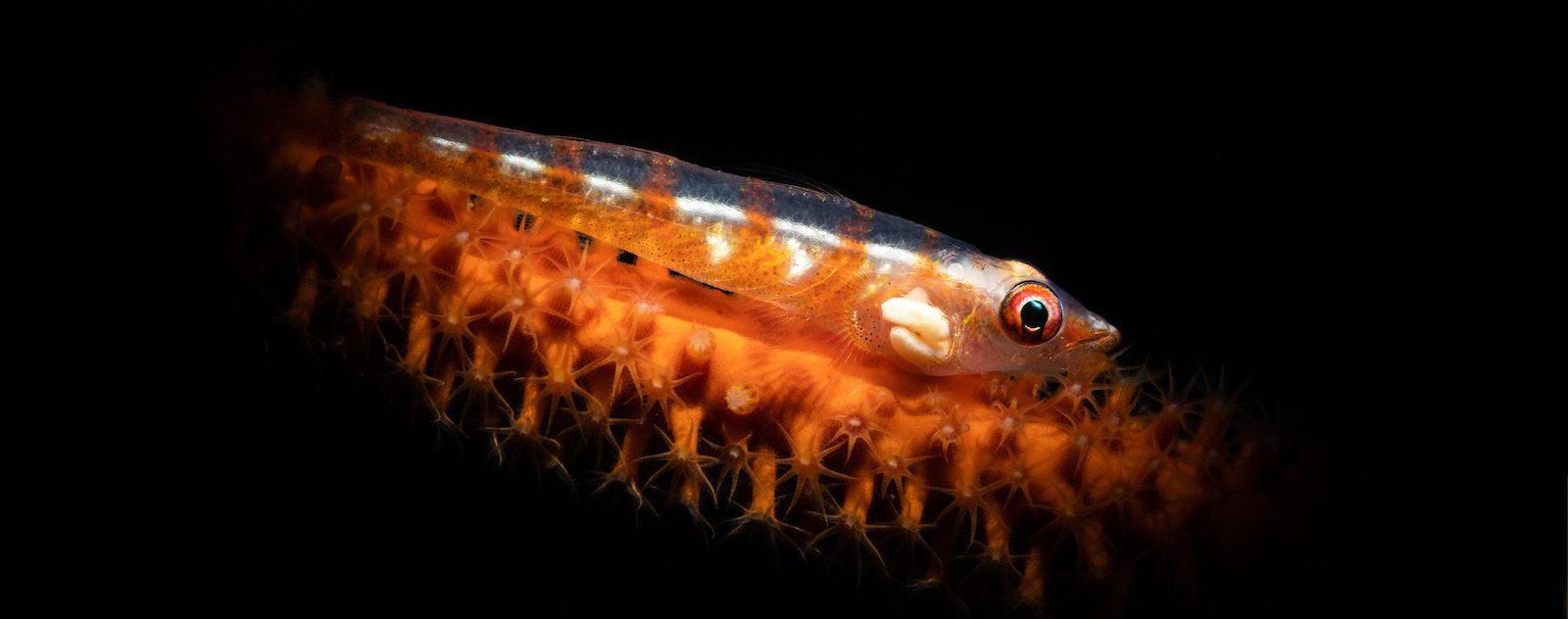This is a close-up color photograph of a small, translucent, silver fish with faint orange stripes running from its head to its tail, totaling eight stripes. The fish has a prominent orange eye with a black pupil and is oriented to the right, revealing internal organs visible through its see-through body, particularly near the gills and fins. The fish is resting on a striking orange, spiky organism, possibly sea vegetation or an anemone-like creature, characterized by numerous spiky protrusions resembling sun shapes. The background is pitch black, giving the impression of the fish and its resting place being spotlighted at the center of the photograph, which creates a dramatic, detailed focus on both the fish and the vividly colored substrate.